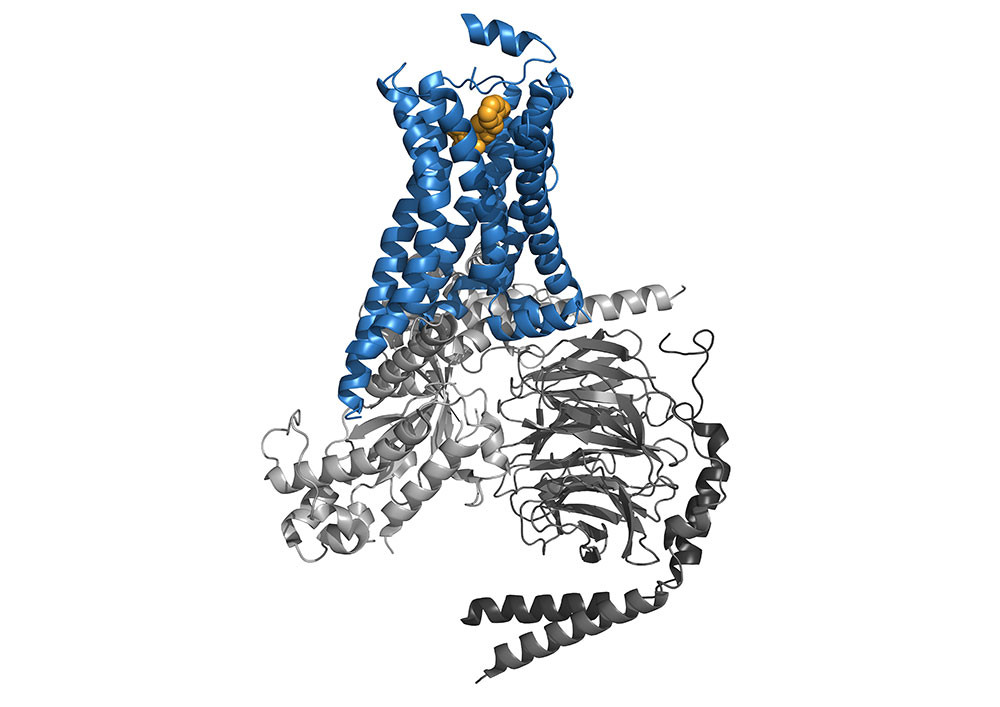This computer-generated image displays an intricate array of spiraled structures akin to party streamers or curly strings, resembling biological or protein models. Scattered across the scene are various color-coded strands: the uppermost grouping primarily features blue spirals interspersed with a cluster of yellow circular shapes at the center. Moving downward, similar spirals in light gray occupy the mid-section, maintaining their tight, curly form. Below these, a pile of dark gray, almost black strands appears stretched out, straightened, and disarrayed, contrasting starkly with the curly shapes above. Finally, at the very bottom, one or two dark gray, nearly black spiral ribbons retain their form, completing the diverse display of twisted and untwisted strands.